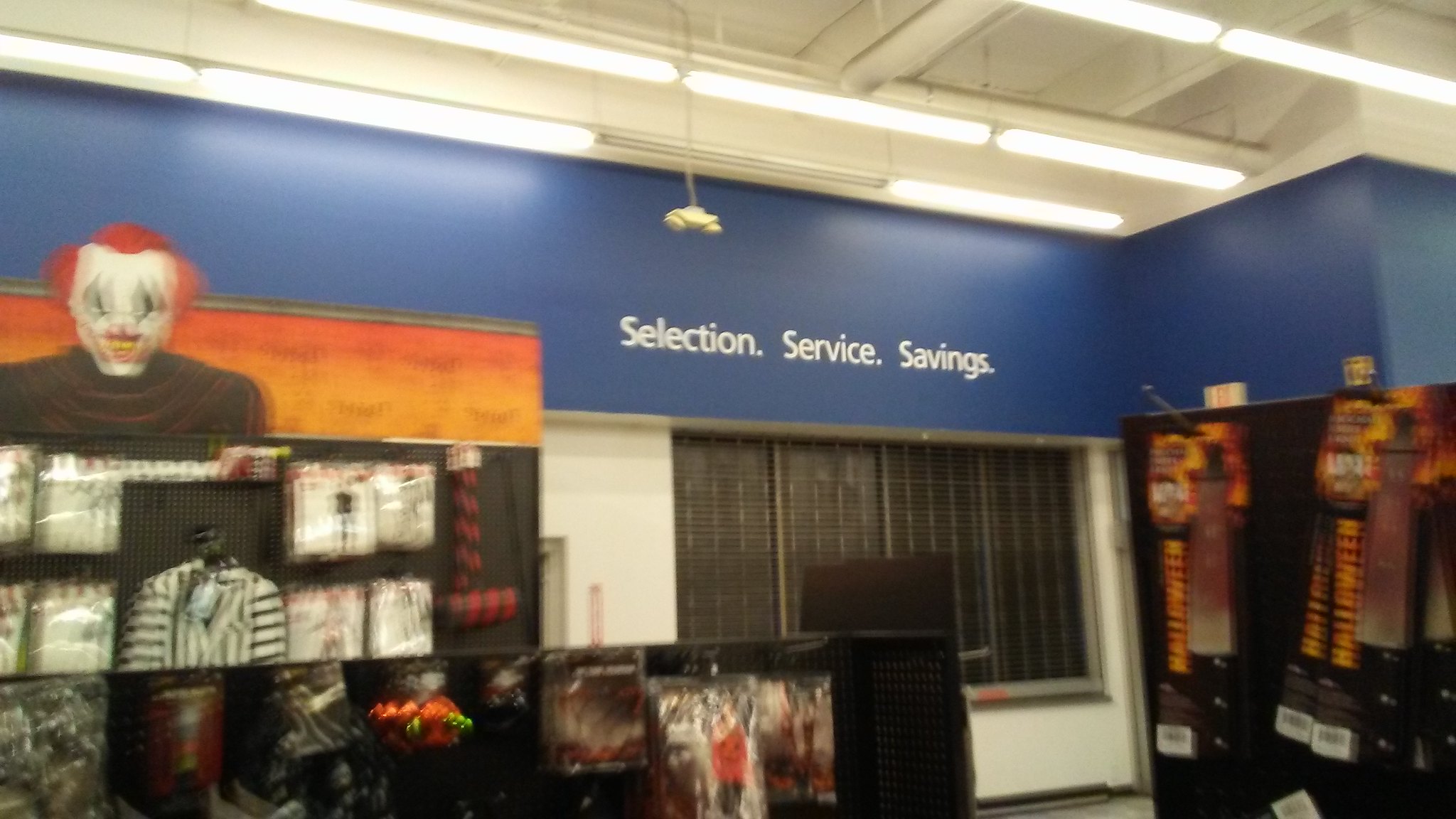This is a blurry color photograph capturing the Halloween section of a store. The store's ceiling is adorned with fluorescent lights, casting a bright glow over the scene. A blue wall in the background prominently displays the words "Selection, Service, Savings" in white lettering. On the left side of the image, there is a display of Halloween costumes, including a noticeable drawing of a demonic clown. To the right, various props are hanging on the wall, though the blurriness makes it difficult to identify them clearly. Among the costumes, a Beetlejuice costume stands out as recognizable. The photograph does not include any people, animals, plants, flowers, or trees. The image has a landscape orientation, being wider than it is tall.